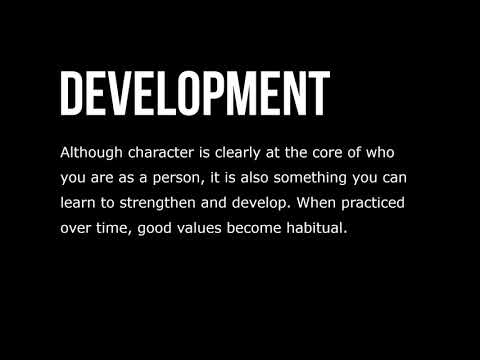The image features a wide rectangular black background with sharp, white text. Positioned slightly left of center and towards the top, the word "Development" is written in large, uppercase letters. Beneath this, in smaller, mixed-case font, a paragraph reads: "Although character is clearly at the core of who you are as a person, it is also something you can learn to strengthen and develop. When practiced over time, good values become habitual." The text is properly punctuated with no grammatical errors, and all elements are spaced evenly within the black background.